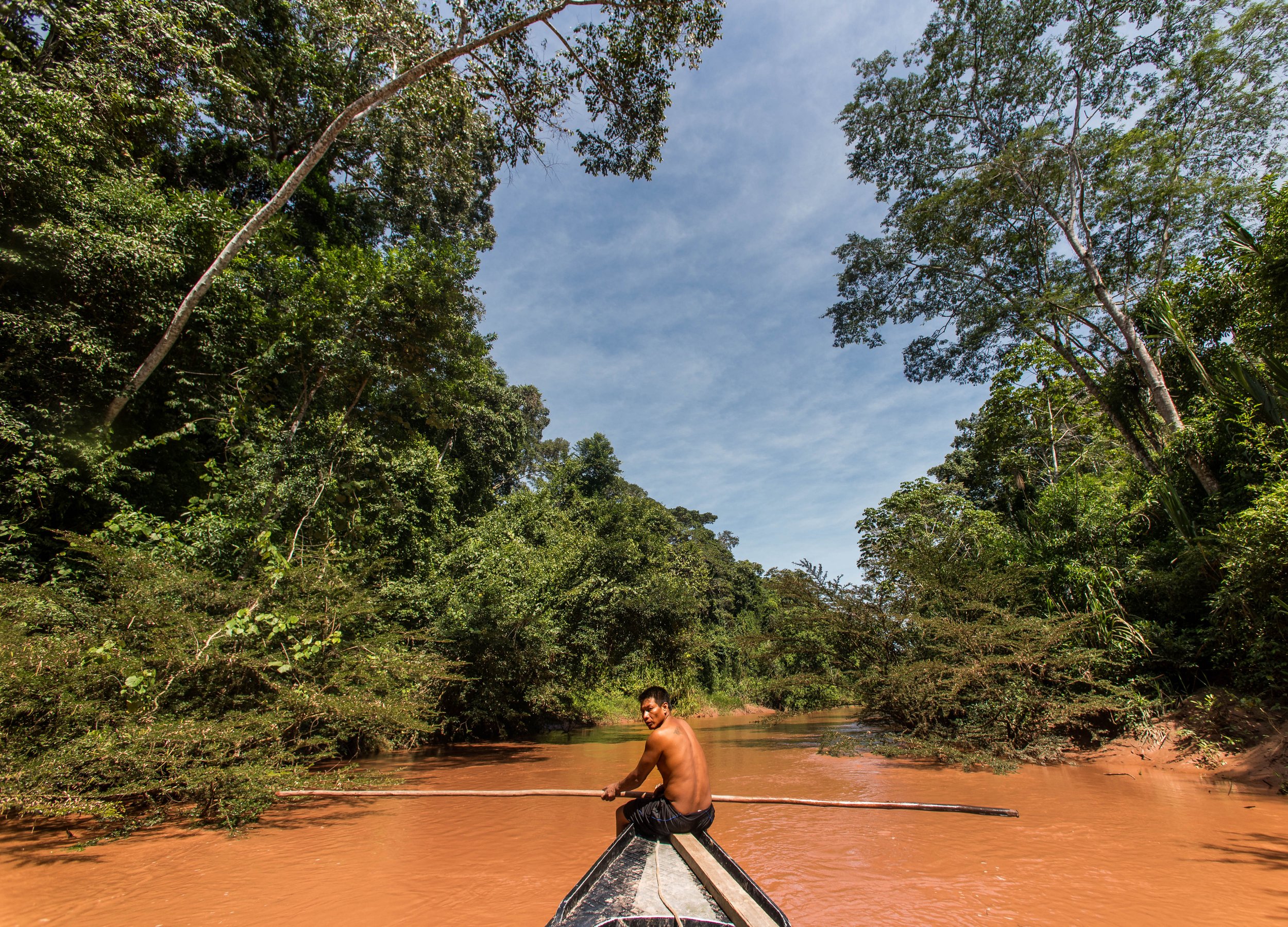A shirtless, tanned man wearing black pants navigates a paddle boat through a vast waterway with a striking orangey-brown, clay-colored hue. The boat, with some black paint worn off, appears to be used for transportation as the man positions himself on a plank at the bow, leveling his seat. He holds a very long pole, twisting back to look towards the photographer, suggesting movement or steering. The water is calm, reflecting its unusual color, while both banks are marked by lush, green vegetation. Some tree branches hang over the water, adding to the scene's greenery. Above, the sky is a bright blue with faint, thin clouds. The setting resembles a large rainforest with towering trees framing the tranquil, clay-colored river, indicating the warm climate.